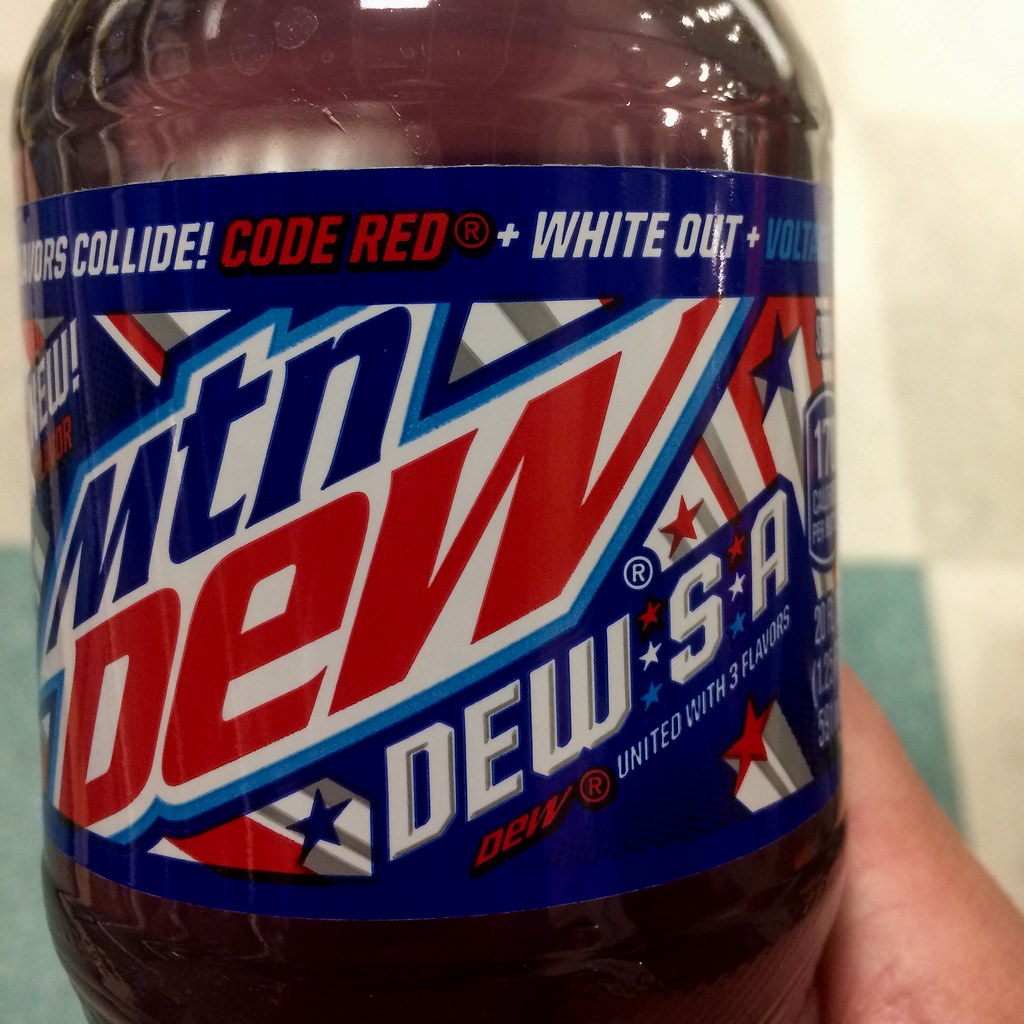The image captures a close-up of a specialty Mountain Dew bottle with a maroon-colored liquid inside. Prominently featured on the label is a blue ring at the top with the text, "Code Red plus White Out plus Voltage" in white. Just below this ring, the recognizable Mountain Dew logo appears, with "Mountain" in blue lettering and "Dew" in red, both set against a white background. This central label is flanked by additional text that curves around the bottle, adding to the visual complexity.

Below the logo, the label reads "Dew S.A." with stars between the "S" and the "A," combining red, white, and blue elements to evoke a patriotic theme. Accompanying this is the phrase, "Dew united with three flavors," indicating a blend of multiple Mountain Dew flavors. Towards the bottom right of the label, a striking red 3D star can be seen, adding to the decorative detail. 

The hand of the person holding the bottle is slightly visible at the bottom right, with a white to lightly tanned skin tone. The background features a floor with white, tan, and teal tiles, adding context to the setting. The bottle reflects a light glare, suggesting overhead lighting, and there is some foam visible just above the label, enhancing the close-up view of this intriguing beverage.